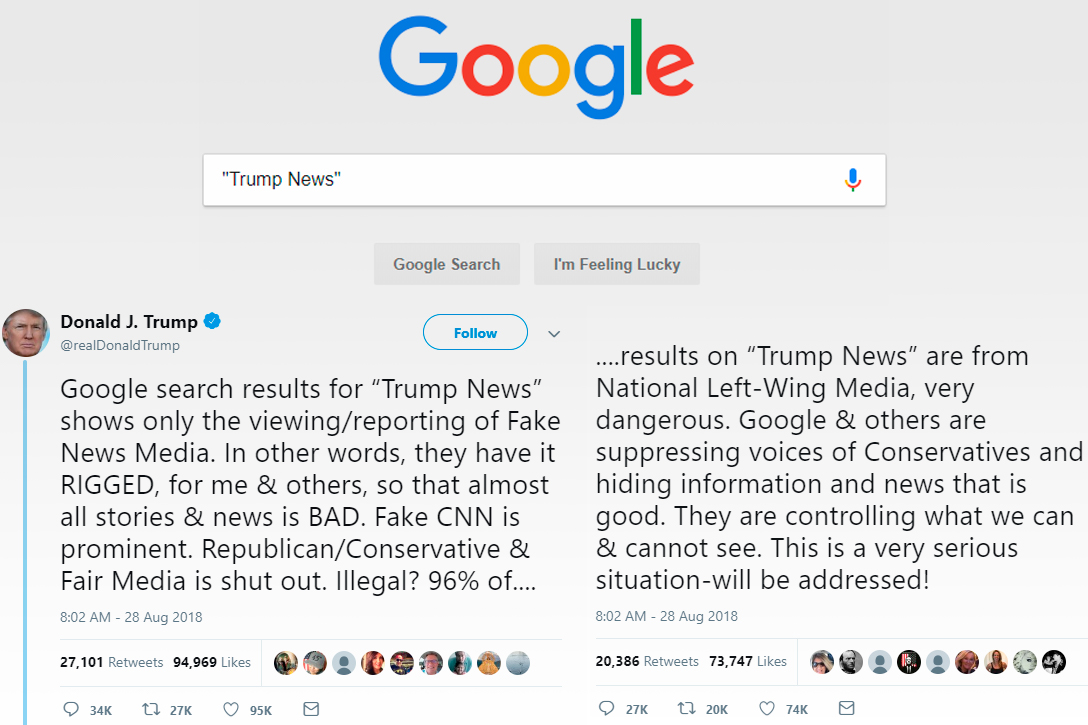The image is a screenshot of a Google search page featuring the familiar Google logo in blue, red, yellow, and green against a gray background. At the top, the search bar displays the query "trump news" in quotation marks, with a microphone icon on the right side. Below the search bar, a profile image of Donald Trump is prominently displayed, accompanied by text that reads "Donald J. Trump" in black lettering, followed by a blue check mark and the handle “@realDonaldTrump.” Next to this is a “Follow” button.

Underneath the profile section is a highlighted tweet by Donald Trump. The tweet reads:

"Google search results for 'Trump News' shows only the viewing/reporting of Fake News Media. In other words, they have it RIGGED, for me & others, so that